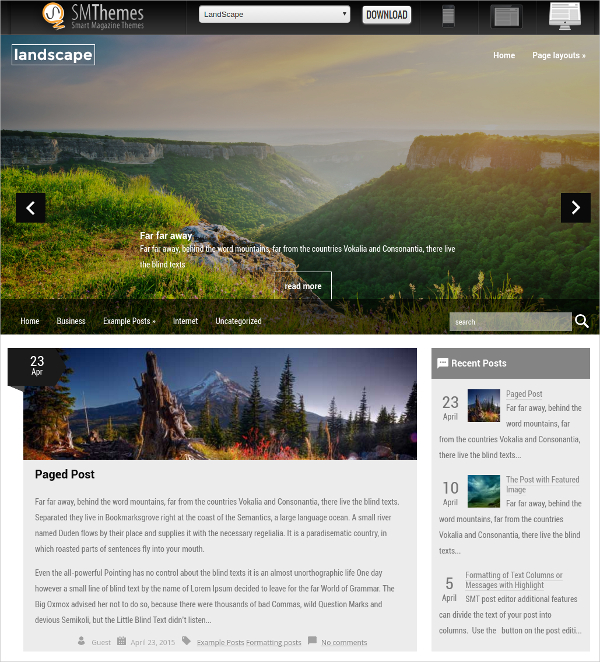This image is a portrait-oriented screenshot of a webpage or design application, approximately one and a half times as tall as it is wide. At the top, there is a black border featuring a logo, which consists of an orange and white circle with a sideways black 'S' in the center. Adjacent to the logo, in gray and white font, the text reads "SM Themes - Smart Magazine Themes."

To the right of the text, there is a gray-colored drop-down box displaying the word "landscape" in black font. Next to this drop-down box is a white rectangular button with prominent black text that says "Download." Below these elements, there are three icons representing different layouts: cellphone, iPad, and computer.

The main section of the screenshot features a landscape image displaying a high-altitude view of mountains, a valley, and a vibrant sky. Overlaid on this image is a white box with the text "Landscape." To the right of this box are navigational options labeled "Home" and "Page Layouts." Near the middle of the image, there are left and right arrows for navigation.

Superimposed on the landscape image in white text is the phrase "Far Far Away," with some smaller, unreadable text beneath it. Below this area, there are transparent border options labeled "Home," "Business," "Sample Post," "Internet," and "Uncategorized."

Finally, at the bottom of the image, there is a box with a background image of a mountain and trees. This box is labeled "Page Posts," accompanied by some additional text. All these elements are set within a gray-colored box.